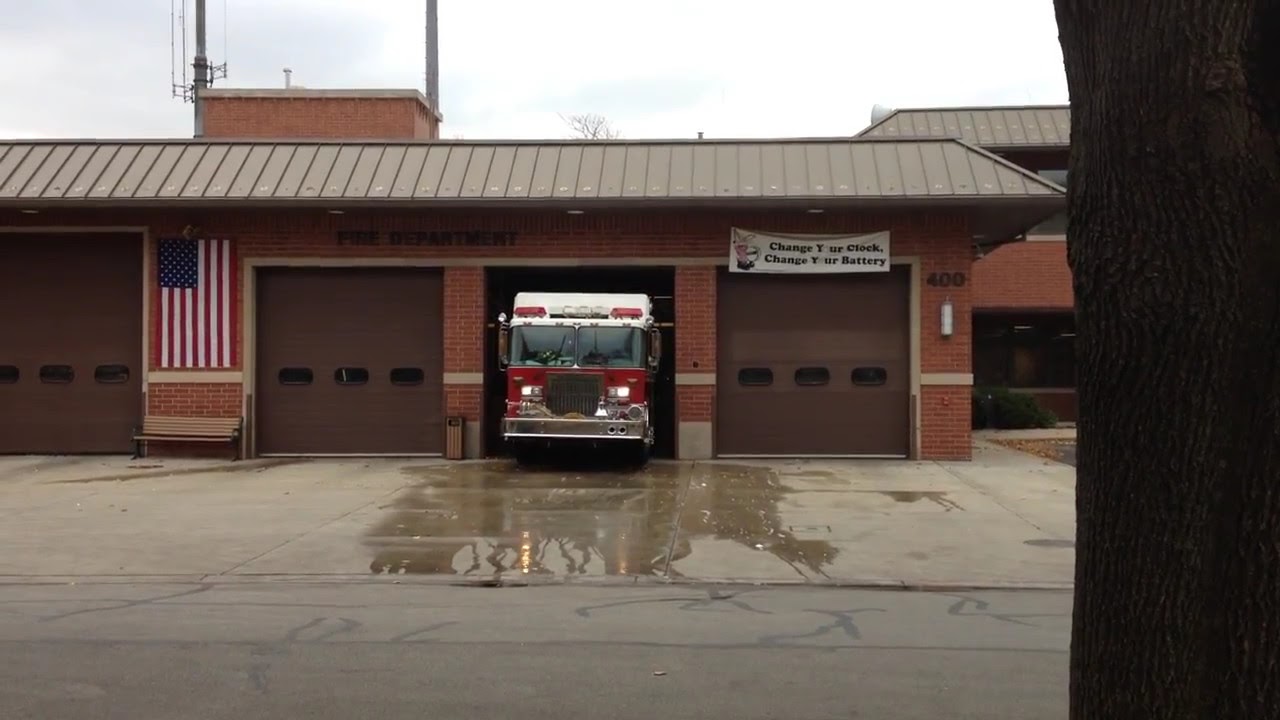This image shows a one-story red brick fire station, distinguished by its address number "400" displayed on the building. The station features four brown garage doors, with three of standard size and one larger one on the left side. The second garage door from the right is open, revealing the front of a fire engine partially emerging. Each of the garage doors has three small windows. Above the far-right garage door, a banner reads, "Change your clock, change your battery," although the white 'O's make the words less visible. Between the third and fourth doors, an American flag is hung vertically on the wall. The building's sloped metal roof and a bench below the flag can also be seen. The words "fire department" are inscribed above the second closed door. In front of the station, water is visible on the driveway, suggesting either recent rain or that the truck is being washed. The scene appears overcast, adding to this possibility. The image is taken from across a cracked and patched light tan street where a tree trunk is visible to the right.